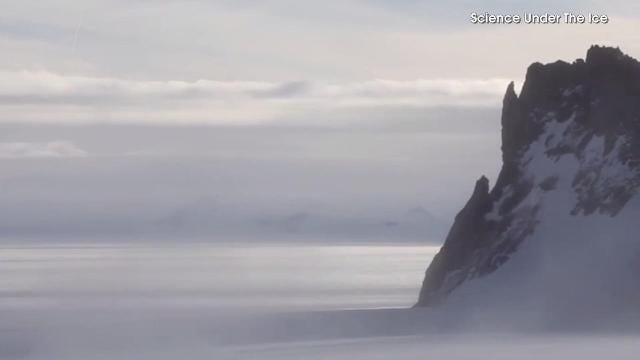This photograph, evocative of a nature program or promotional image, captures a stark and cold outdoor scene dominated by elements of snow, ice, and rugged terrain. In the upper right-hand corner, "Science Under the Ice" is prominently displayed in white text with a black border. The landscape is a blend of thick, white clouds that seem to descend into layered colors of grays and blues, merging seamlessly with the snow-covered ground. The right side of the image features a rugged, mountainous outcropping, partially cloaked in snow and bearing a dark brown, rocky surface. The overall atmosphere is one of harsh, wintry desolation, with a sky that is almost completely white, enhancing the sense of coldness and isolation.